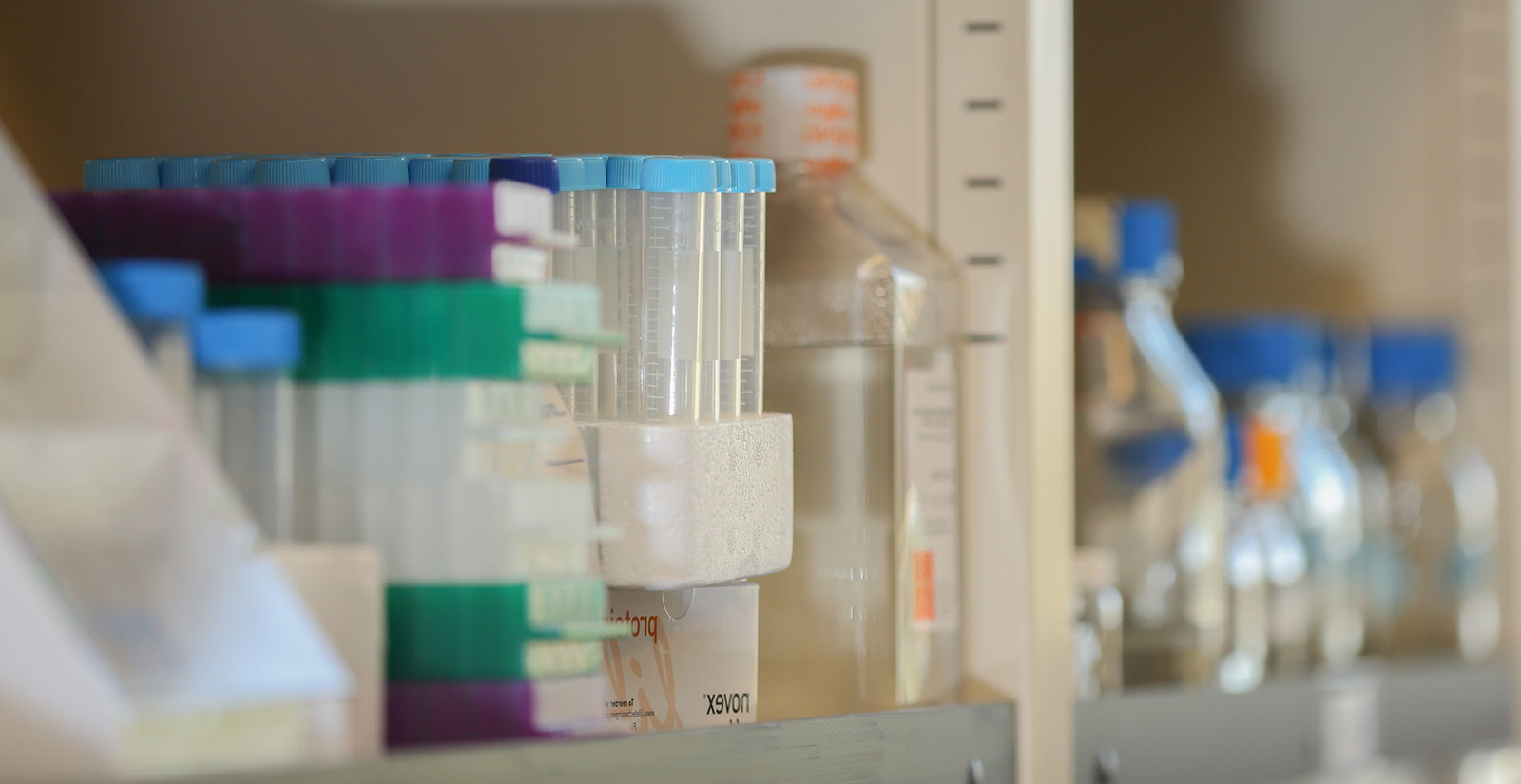A shelf in a medical facility is meticulously organized with various laboratory supplies. On the left side, several white bins hold clear test tubes, each featuring a white labeling strip and measurement markings, topped with light blue caps. Adjacent to these bins, there is a somewhat blurry stack comprising green, purple, and white objects, though their exact nature is indistinguishable. Nearby, additional test tubes are stored alongside a clear bottle sealed with an orange cap and a white lid, placed on off-white shelving units. The adjacent shelf holds a collection of glass jars capped with blue tops, with a hint of orange visible among them, though its exact details are obscured by the blur. The overall setup indicates a well-maintained laboratory environment, equipped for precise scientific work.